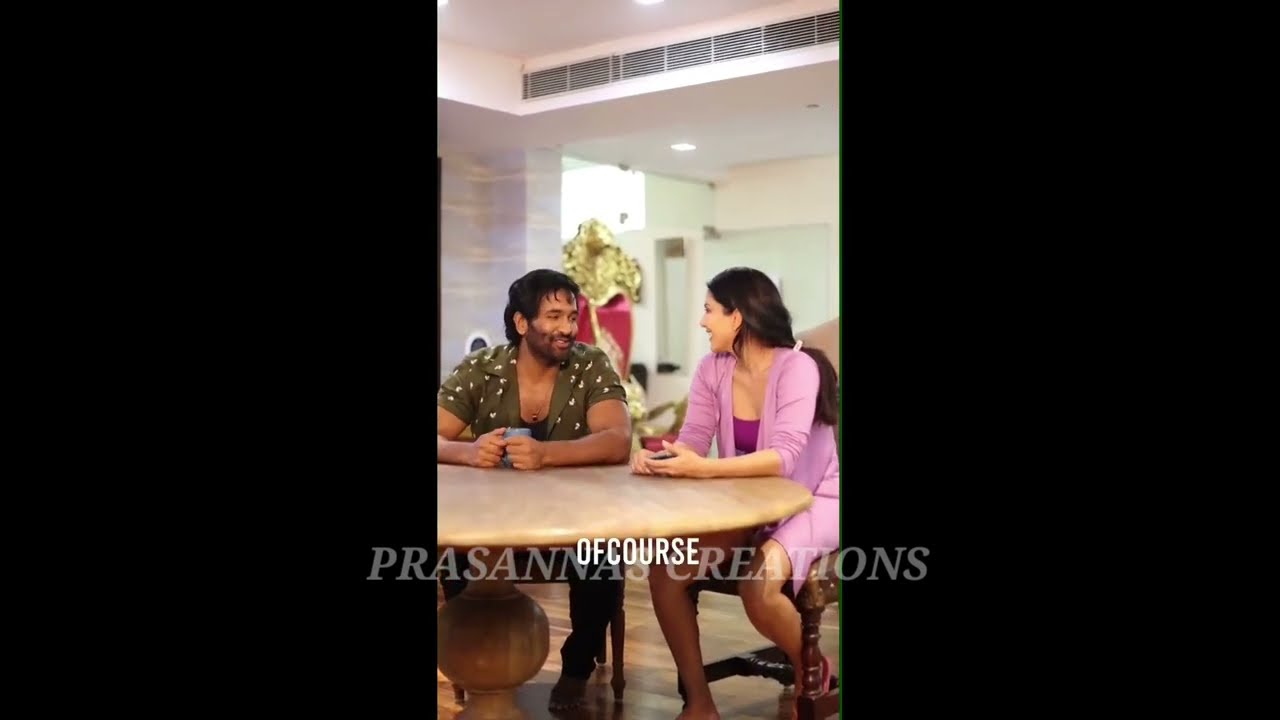The image is divided into three equal rectangles, with the left and right sections completely black, and the central rectangle containing a detailed picture of a couple seated at a round wooden table in a spacious room with white walls and a light brown wooden floor. The man, positioned on the left, has slightly darker brown skin, dark hair that's a bit longer at the back, and a neatly trimmed beard and mustache. He wears an open dark moss green shirt with white dots over a black tank top and possibly a necklace, and holds a blue mug. His elbows rest on the table as he looks at the woman. The woman, seated on the right, has light brown skin and long, darker brown hair pulled back into a low ponytail. She wears a light pink long-sleeved sweater over a dark pink tank top and appears to be holding a cell phone. Both individuals are looking at each other, engaged in a moment. Overlaying the image in faint font are the words "personas creations," with "of course" in a bolder white font superimposed over it.